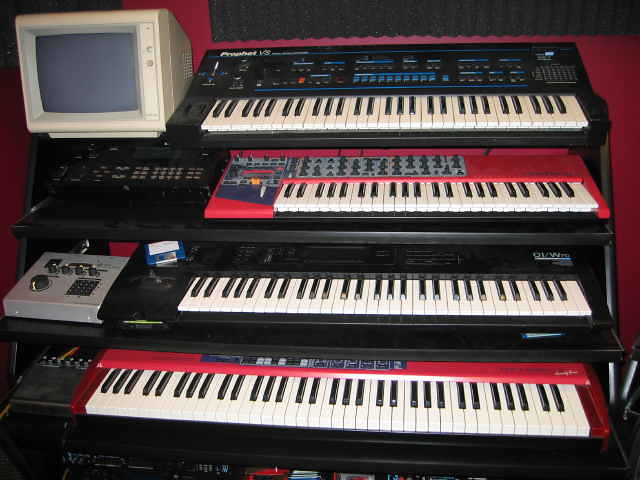The photograph depicts a room with red walls containing a shelving unit that holds four electronic piano keyboards arranged vertically. The top keyboard is black and features red buttons. To the left of this keyboard, there is an old-fashioned CRT computer monitor. The second keyboard from the top is red with black controls. Below it is a black keyboard with black controls. The bottom keyboard is red with gray controls and is the longest of the four. There is also a blue floppy disk on one of the keyboards. Below the keyboards, the shelving unit holds audio equipment, including devices with various buttons and knobs for sound manipulation and possibly an old speaker. The equipment and overall setup give the room a vintage feel, reminiscent of the 1990s.